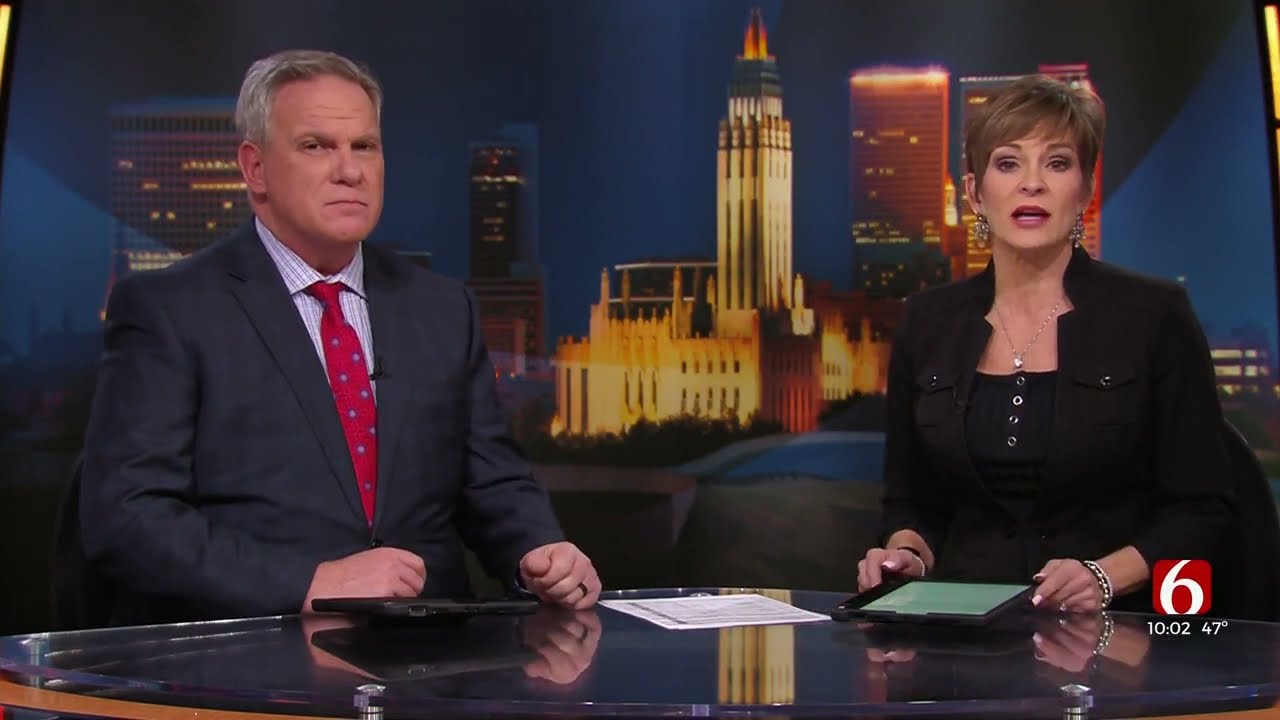The image is a screenshot from a nightly local newscast on Channel 6, identifiable by the lower right-hand corner logo—a white "6" on a red background, along with the time "10:02" and temperature "47 degrees" in white text. Seated at the news desk are two anchors: a Caucasian male on the left and a Caucasian female on the right. The male anchor, with short gray hair and a high forehead, is dressed in a dark gray suit with a red tie featuring a dotted pattern, paired with a light blue button-down shirt. His arms rest on the shiny, reflective surface of the desk. The female anchor, with short brown hair styled close around the sides and bangs on her forehead, is wearing a dark scalloped lapel jacket over a low-cut black blouse with central buttons. Her sleeves are pushed up slightly above her wrists. She is holding a green-screened tablet between her hands, positioned on the reflective desk alongside a flat piece of white paper. Both anchors are looking directly into the camera, with the female anchor appearing to speak, her mouth slightly open, while the male anchor’s mouth remains closed. Behind them is a classic nighttime cityscape backdrop, reflected on the clear surface of their desk, adding to the professional news atmosphere.